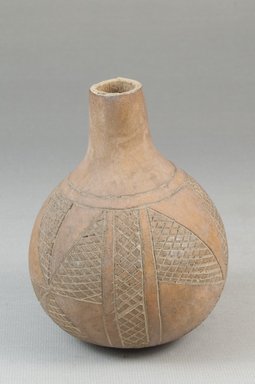This image showcases an ancient artifact, a clay pot, displayed in a gallery setting against a smooth, grey, featureless background. The pot, possibly carved from a gourd, features a bulbous, spherical body roughly the size of a child's basketball. It tapers into a small, tubular neck with an opening that's significantly larger than a bottle's but still relatively narrow. The neck appears sawed off at the top, creating a distinctive sliced-off effect. The exterior of the pot is adorned with intricate etchings that form a grid-like or diamond-patterned design, divided into geometric sections such as stripes and triangles. The pottery has a matte finish and a pinkish hue, enhancing its artifact-like appearance. The meticulous engravings resemble a series of tiles, flags, and columns, giving the pot both an artistic and historical significance.